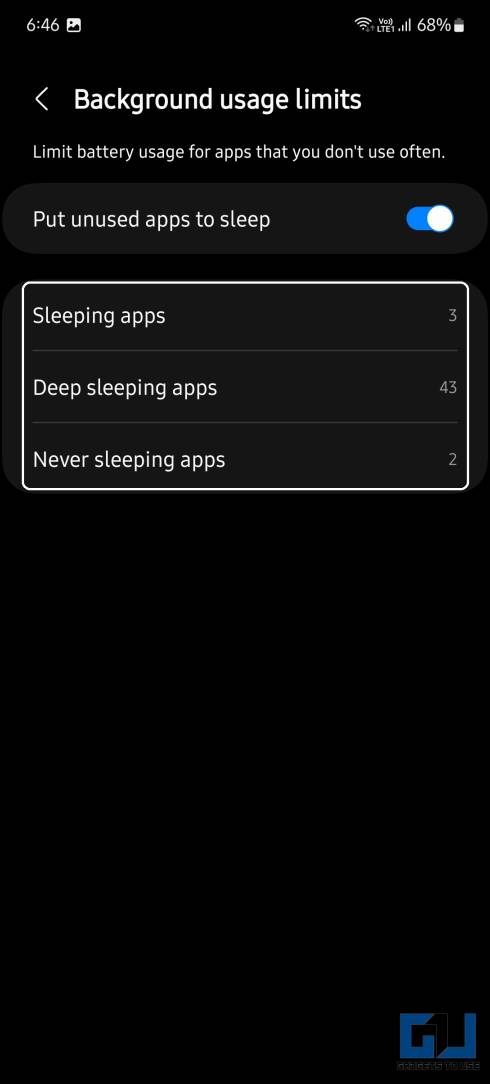The screenshot displays a cell phone screen with various indicators and settings. In the upper left-hand corner, the time reads "6:46". In the upper right-hand corner, there is an image of a wireless signal icon followed by "LTE" and four bars, indicating strong cellular connection strength. Next to this, the battery status shows "68%" with a mostly full battery icon.

The background of the page is black, and all text on it is in white, creating a high contrast. Prominently displayed across the top in larger print is the phrase "Background usage limits." Below this, in smaller text, it explains the function: "Limit battery usage for apps that you don't use often." Beneath this descriptive text, the phrase "Put unused apps to sleep" is visible and this option is selected. 

Further down, there is a white-bordered rectangle containing the text "Sleeping apps." To the far right of this text, the number three is displayed, indicating the number of apps in this category. Below that, "Deep sleeping apps" is listed, with the number 43 on the far right. Continuing down, the text "Never sleeping apps" appears, accompanied by the number two on the far right. 

A large area of the black background with no text follows, and in the lower right-hand corner of the page, the initials "GJ" are inscribed in blue.